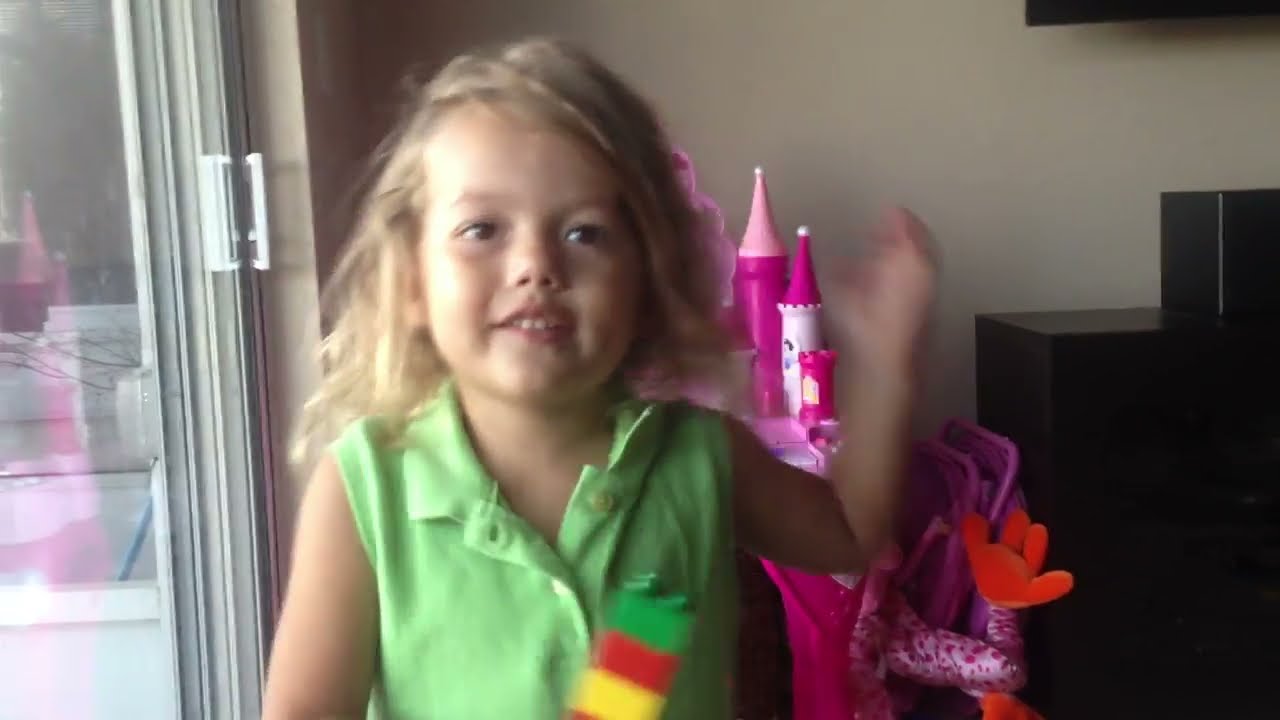The image depicts a small girl, likely about four years old, standing in the center of a toy-filled room. She has light brown, somewhat messy, shoulder-length hair that is parted on the side. Her expressive brown eyes and soft brown eyebrows frame a pudgy nose. She is dressed in a lime green sleeveless top. The girl is holding a stack of colorful Duplo blocks with her right hand, lifting them to her mouth as if she is pretending to play them like a horn. Her left arm hangs naturally by her side. In the background, a pink princess castle that seems to double as a vanity, complete with various shades of pink and a hint of white, stands to her left. To her right, there is a Disney-themed blue toy box featuring Ariel from The Little Mermaid, accompanied by Flounder. A white stuffed animal, resembling a dog, lies on the floor in front of the toy box. Behind her, a black entertainment stand that appears to house electronic equipment is visible, along with part of a black TV mounted above it. The wall behind the girl is painted a light tan color, adding a neutral backdrop to the playful scene.